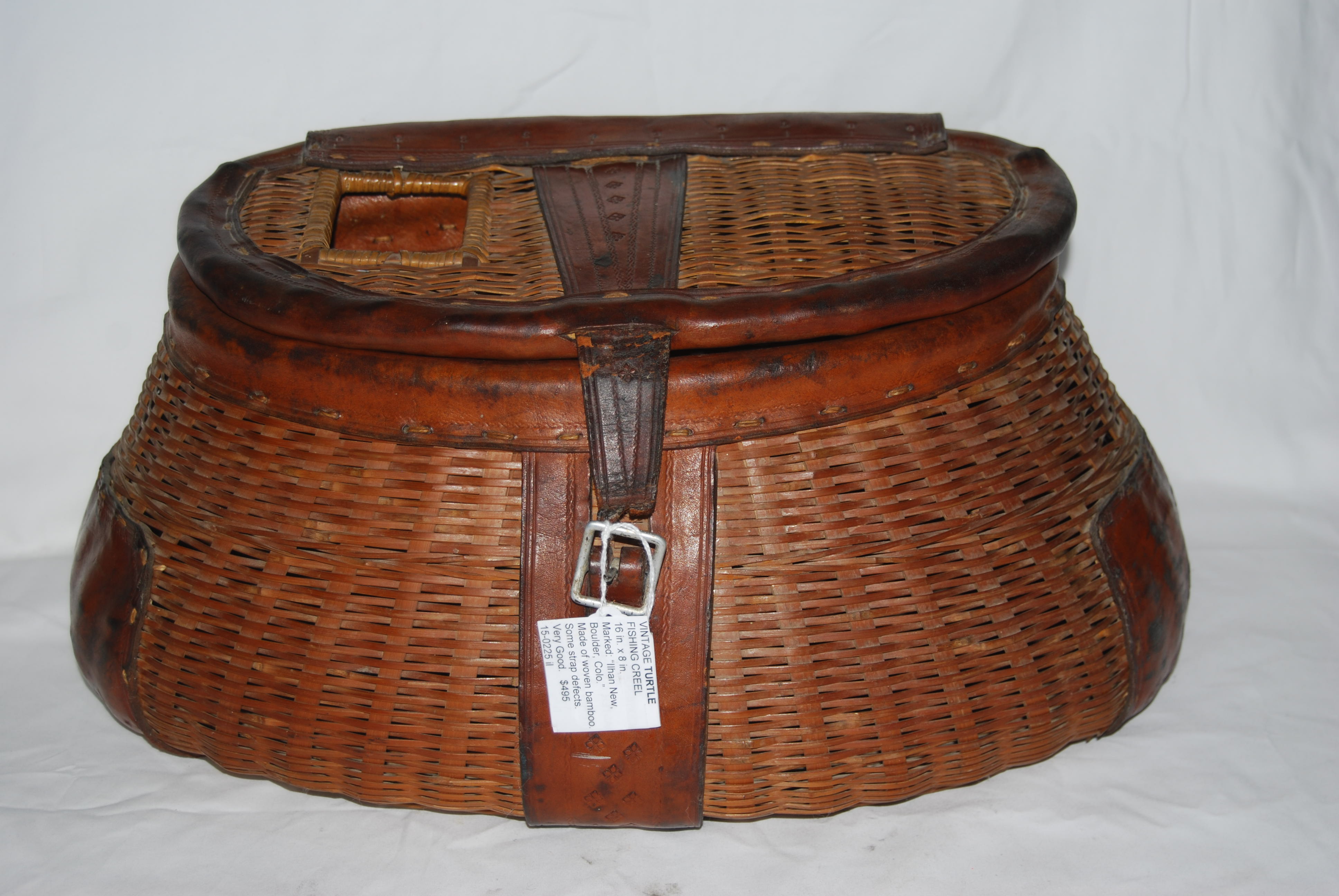This detailed photograph showcases a vintage wicker fishing creel, skillfully woven from bamboo, presented on a white fabric background. This dark brown basket, measuring 16 inches by 8 inches, features a distinct oval shape with slightly triangular sides. The basket is secured by a front leather strap that latches with a silver buckle. Attached to the buckle is a white tag inscribed with "Vintage Turtle Fishing Creel 16x8," and additional text indicating it's priced at $495. The creel, in very good condition, displays a harmonious blend of light to dark brown hues, with the wicker weaving displaying subtle reflections of light. The leather components and edges, including a triangular strap and rounded borders, add to the vintage charm of this well-preserved piece of fishing history.